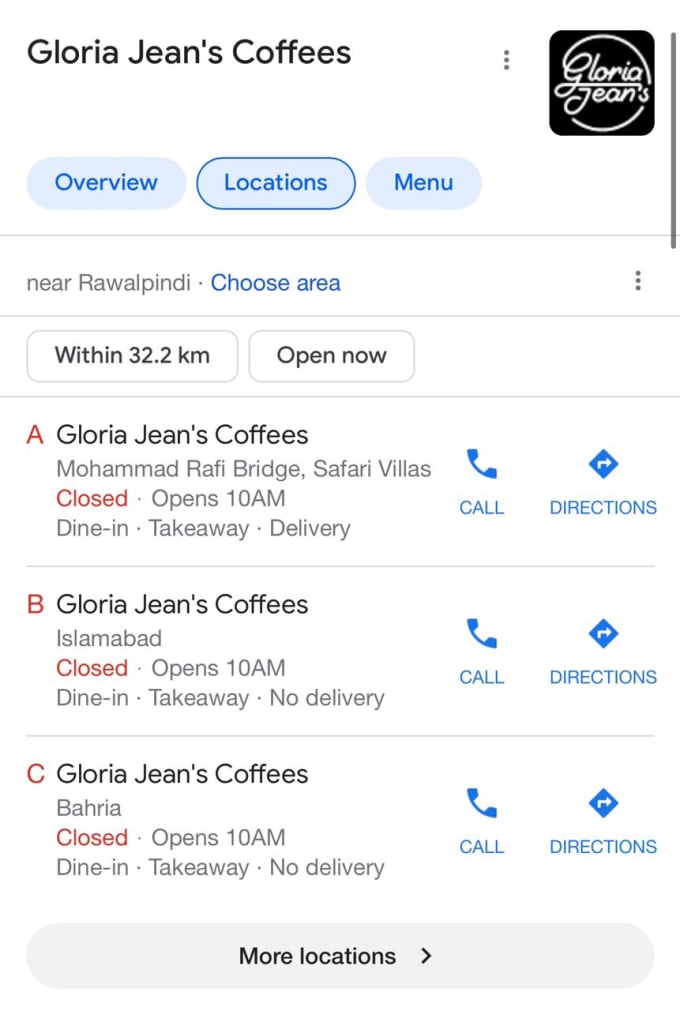The image depicts a Google search result for "Gloria Jeans Coffees." At the top of the search results, the headline reads "Gloria Jeans Coffees," accompanied by the store's logo on the right. The logo features the text "Gloria Jeans" with "Gloria" on top and "Jeans" on the bottom, all enclosed in a large circle. The text is white set against a black background. 

The Google search interface itself has a white background. Below the headline and logo, the categories "Overview," "Locations," and "Menu" are listed, with "Locations" selected. The search specifies locations near Rawalpindi. 

Three specific Gloria Jeans Coffees locations are detailed:
- **Location A:** Gloria Jeans Coffees at Muhammad Rafi Bridge, Safari Villas. The status shows "Closed, opens 10 a.m." It offers options for dine-in, take-out, and delivery. The entry includes icons for calling the location and getting directions.
- **Location B:** Gloria Jeans Coffees in Islamabad. This location is also "Closed, opens 10 a.m." Availability includes dine-in and take-away, with no delivery option. It similarly includes call and directions icons.
- **Location C:** Gloria Jeans Coffees in Bahria. Like the others, it is "Closed, opens 10 a.m." and provides dine-in and take-away services without delivery. Call and directions icons are also present.

Below these entries, a gray button with black text reads "More Locations," suggesting the user can click to find additional Gloria Jeans Coffees locations.